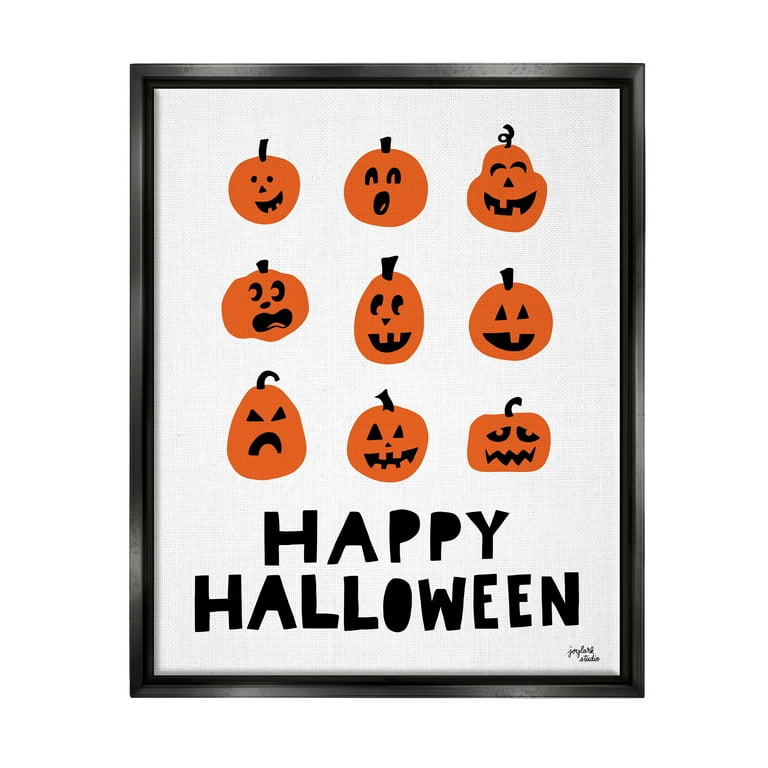The image features a festive Halloween-themed illustration enclosed in a black frame. Set against a white background, the artwork displays twelve orange pumpkins, each carved with unique expressions ranging from happy and smiley to scary and shocked. The faces and stems of the pumpkins are rendered in black. Below these pumpkins, "Happy Halloween" is written in bold black letters, adding a celebratory touch to the piece. In the bottom right corner, there's an artist's signature in small cursive, though it's difficult to discern. This canvas print, with its detailed texture, is ideally suited for bringing a festive Halloween spirit to any home or business.